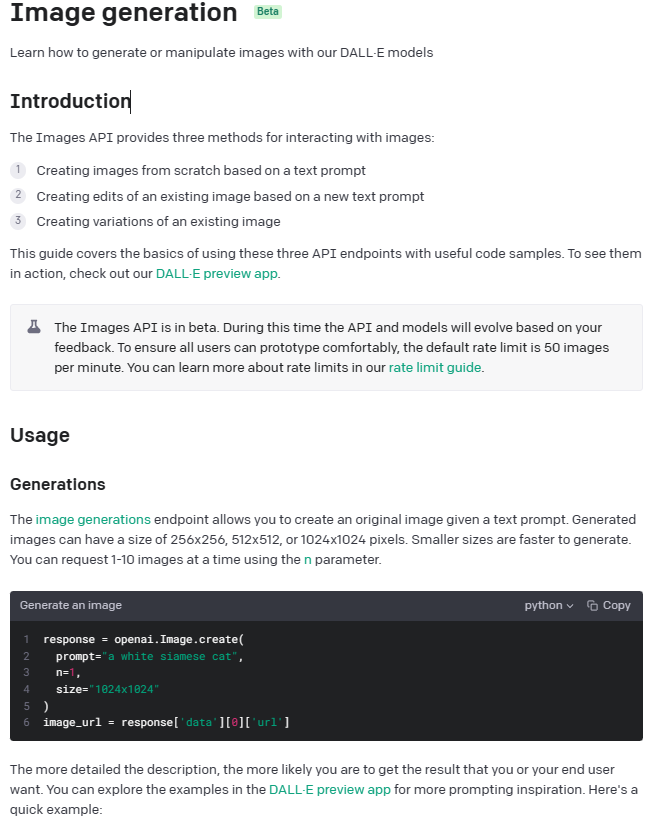**Detailed Image Caption:**

_DAO-E Image Generation Guide_

Explore the innovative capabilities of image creation and manipulation with our DAO-E models, currently in Beta. This guide introduces the three primary methods for interacting with images via our API:

1. **Creating Images from Scratch**: Utilize text prompts to generate entirely new images.
2. **Editing Existing Images**: Modify an existing image based on a new text prompt.
3. **Creating Image Variations**: Produce different versions of an existing image.

This comprehensive guide provides an overview of these three API endpoints, complete with useful code samples. For a hands-on experience, visit our DAO-E preview app. Note that the Images API, being in beta, will undergo continual enhancements driven by user feedback. To facilitate smooth prototyping for all users, the default rate limit is set at 50 images per minute. Further details about rate limits can be found in our dedicated guide.

**Usage Generations**:
Leverage the image generations endpoint to create original images from text prompts. Generated images come in three sizes: 256x256, 512x512, or 1024x1024 pixels, with smaller sizes generating faster. You can request between 1 to 10 images at a time via the 'end' parameter. 

_Example code snippet:_ Generate an image using Python.

This guide is your gateway to mastering image generation and manipulation using DAO-E's powerful models, empowering your creative and technical endeavors.